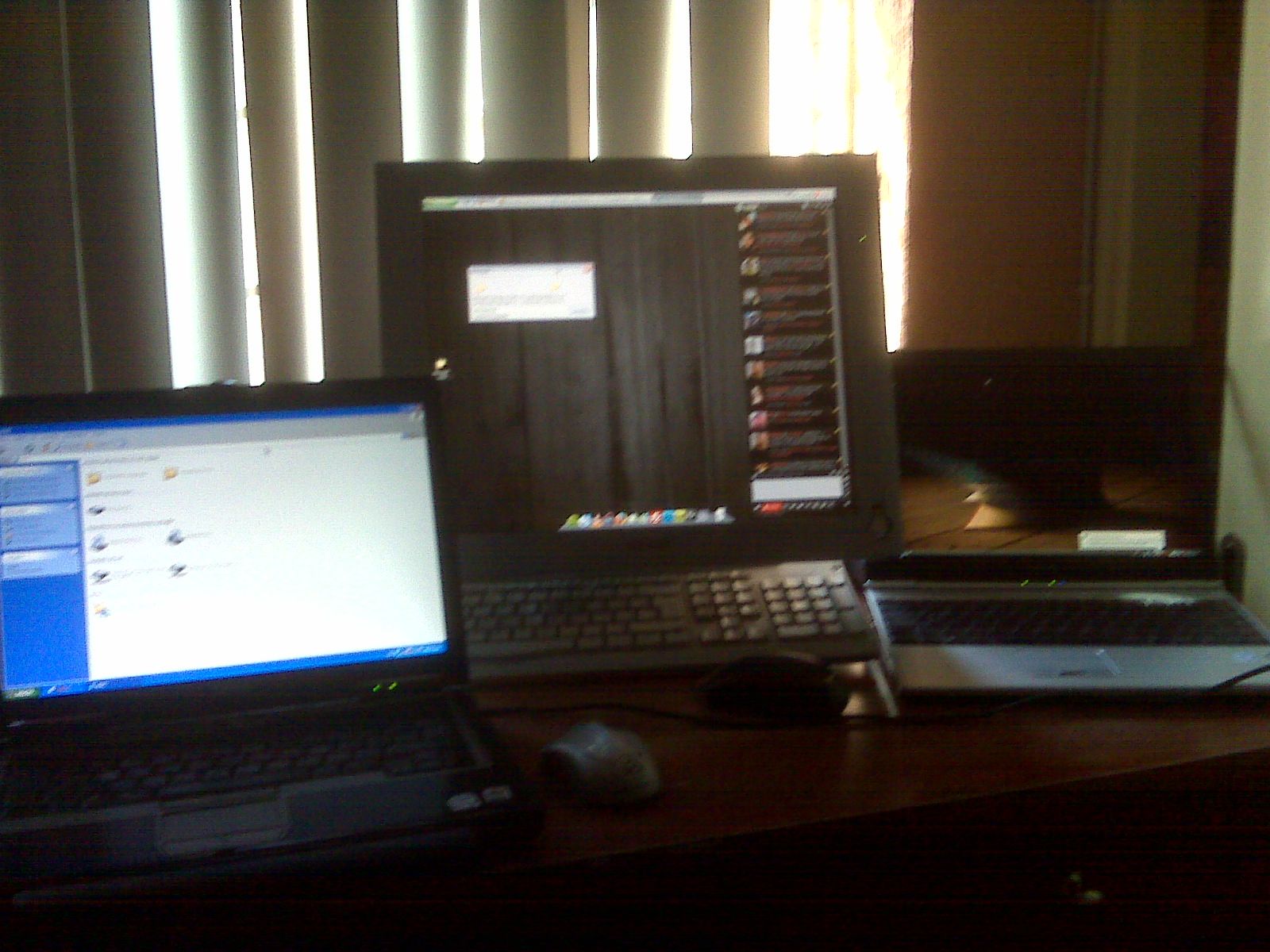The image is a blurry, color photo from the early 2000s, taken inside a poorly lit room with vertical blinds partially turned to block the light, although some sunlight still pours through. The room appears to be a hotel room, given its nondescript nature and standard furnishings. The focal point is a dark wooden desk or table placed in front of a large window or sliding glass door. On the desk, there are three devices. 

On the left, there's a laptop powered on and displaying the Windows XP file manager screen with a white background and a bright blue border. In the center, there is likely an old Mac device, possibly an iMac, adding to the dated feel with its all-in-one design, though the screen's content is indistinguishable due to the blur. On the right side, another open laptop is visible, suspected to be running Windows Vista given its gray taskbar, but it’s hard to confirm if it's powered on or simply reflecting the surroundings. Despite the graininess and poor focus, it’s also evident that separate wireless mice accompany at least two of these devices.